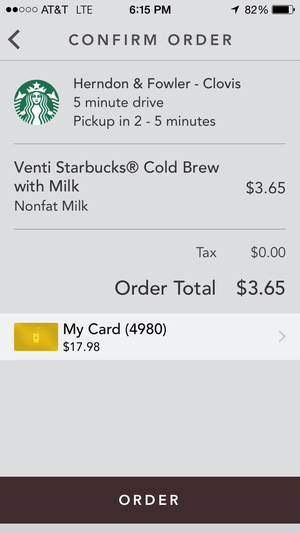This image is a detailed screenshot from a mobile phone. At the very top, the background is grey, featuring status indicators including two black dots and three empty dots. The status bar displays "AT&T, LTE," and the time, "6:15pm." Location sharing is enabled, and the battery level is shown at 82%, accompanied by a corresponding icon.

Below the status bar, there is a grey screen with black text that reads "Confirm Order." An icon of the Starbucks logo, depicting a woman with a crown and long flowing hair, is prominently displayed. The text next to the icon reads "Herndon and Fowler-Clovis, 5 minute drive, pick up in 2-5 minutes."

Further down, the order details are listed:
- "Venti Starbucks Cold Brew with Milk, Nonfat Milk"
- Price: "$3.65"
- Tax: "$0.00"
- Total: "$3.65"

Below the order details, an icon of an orange credit card is shown with the text "My Card 4980," indicating the last four digits of the credit card being used for the purchase. The available balance on the card is "$17.98."

The bottom section of the screenshot features a black rectangular button with the word "Order" written in white font.